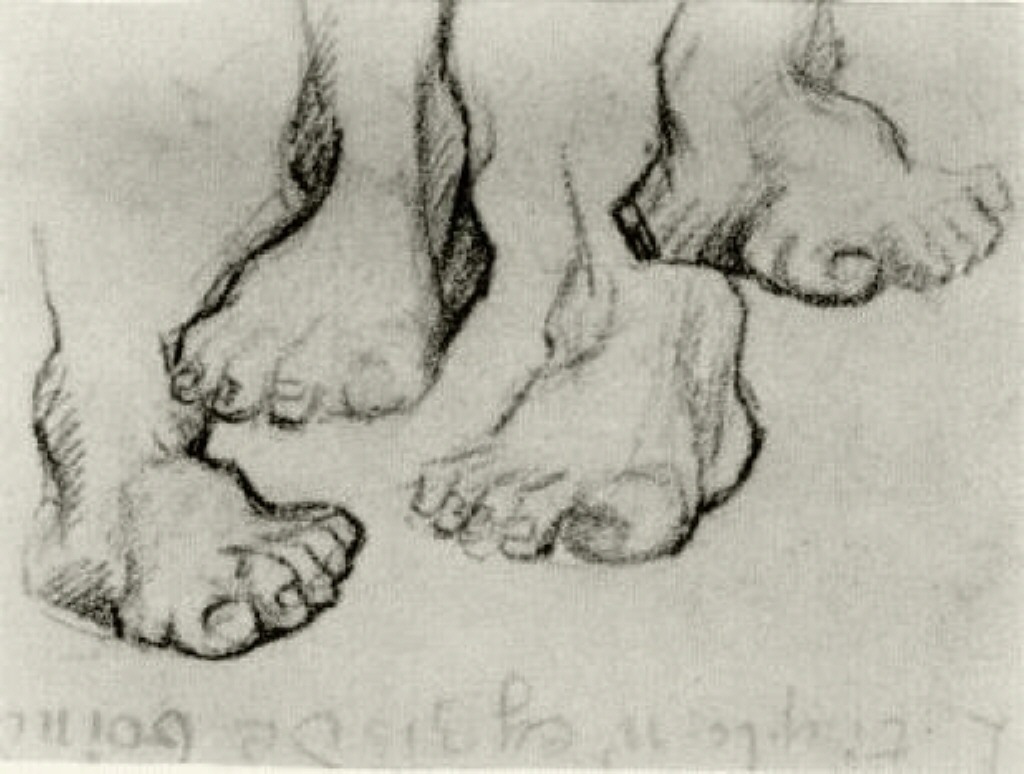The image is a hand-drawn sketch set on aged, off-white or grey paper, depicting four detailed and burly feet, each with short nails and chunky toes. The feet, two left and two right, vary in orientation: the leftmost foot points to the right, the second foot points towards the bottom left, the third foot also points to the bottom left but is turned more to the left, and the rightmost foot points to the right. In the center of the image, there is some faint text that is hard to decipher, appearing to be in a non-English language and possibly reversed and upside down. The sketch emphasizes the thick, muscular nature of the feet, making them appear lumpy yet robust.